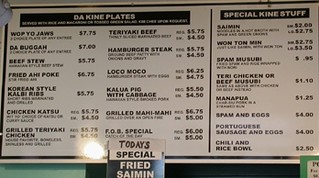In this close-up image of a menu, the small size and resolution make it somewhat challenging to read. The bottom part of the menu reveals a portion of a green-painted wall and a black strip that appears to be part of a doorway. In the bottom right corner, there's a partially visible sign, but the text on it remains unreadable. The bottom of the menu features the heading "Today's Special," which is listed in black and white text and reads "Fried Salmon." Above this are various menu categories and items. The "Plates" section includes dishes such as "Korean Style Ribs," "Chicken Katsu," "Grilled Teriyaki Chicken," "Teriyaki Beef," "Loco Moco," "Hamburger Steak," and "Kalua Pig with Cabbage." On the right side, another category titled "Special King Stuff" lists items like "Salmon" and "Spam and Eggs."